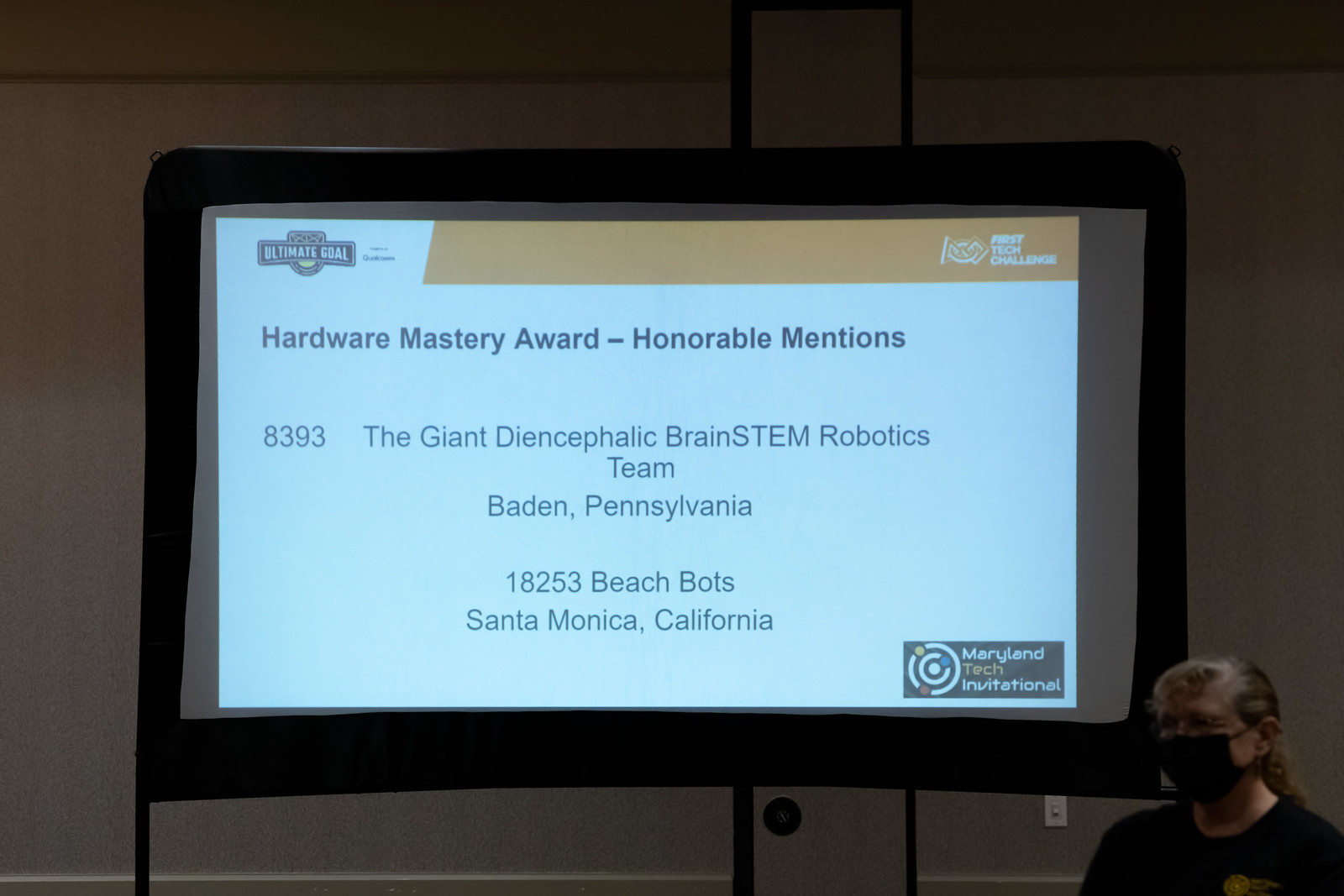The image depicts a large projection screen with a black border, occupying the majority of the frame, suggesting a conference or event setting. The screen displays what appears to be a PowerPoint slide under a white background. At the top-left corner, the screen features a logo with the text "Ultimate Goal." An orange bar spans across the top portion of the slide, with some unreadable white text to the top-right. Below the bar, the title "Hardware Mastery Award - Honorable Mentions" is prominently displayed. Beneath this, there is a sequence of text elements: "8393" on the left, followed by "The Giant Diencephalic Brainstem Robotics Team, Baden, Pennsylvania," and an address in Santa Monica, California including "18253 Beach Bots." Towards the bottom-right of the screen, the text reads "Maryland Tech Invitational," accompanied by a small diagram of an atom. In the lower right corner of the image stands a woman, partially visible, wearing a black COVID mask, a black T-shirt, and glasses. She has gray hair, presumably tied back, and is facing forward. Her figure is cropped at the chest by the bottom edge of the image, indicating that the photo captures her presenting or attending the event.